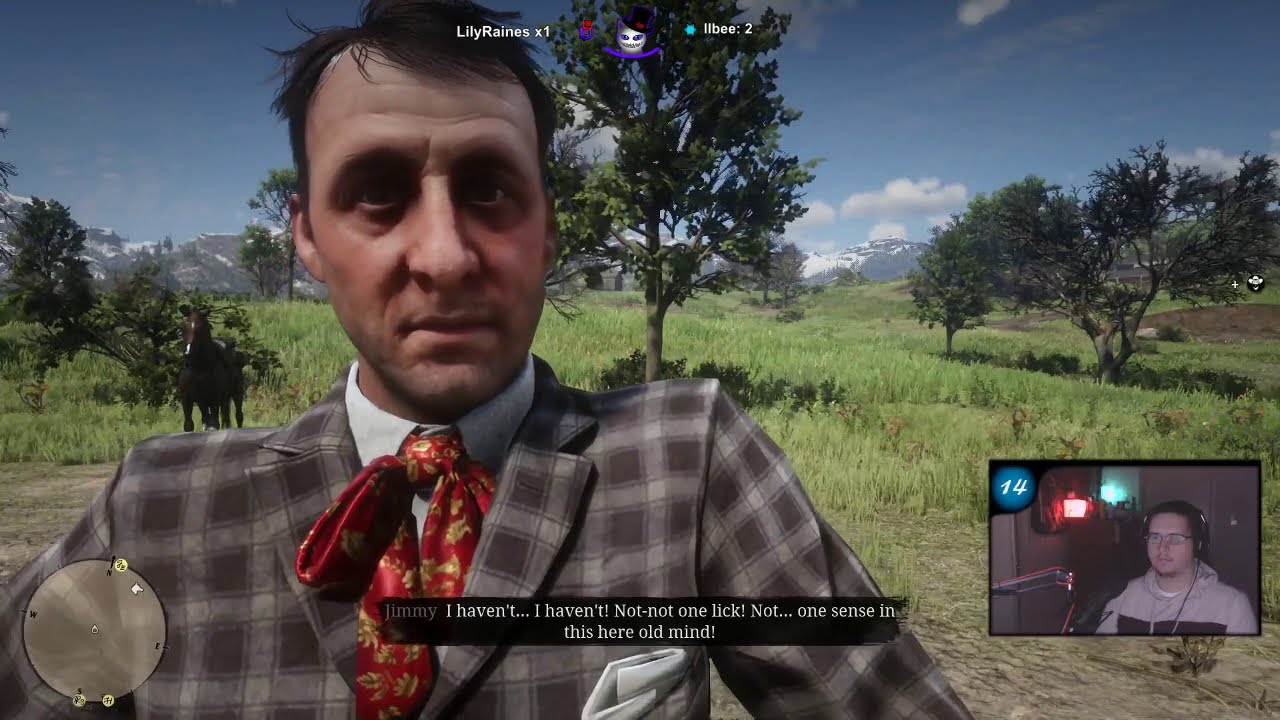The image is a detailed screenshot from what appears to be the video game Red Dead Redemption 2, captured while being streamed online. Dominating the left-center of the image is a middle-aged white man with short, sparse dark hair, and a somewhat frowning expression. He is dressed in a checkered suit, primarily in shades of brown, gray, and off-white, paired with a distinctive red bow tie decorated with gold, and a crisp white collared shirt. A white handkerchief peeks out from his blazer pocket. Behind him, a picturesque landscape unfolds, featuring tall green grass, several blooming trees, and a brown horse in the mid-ground, all set against a backdrop of a mountain range topped with patches of snow and a partly cloudy blue sky.

Toward the top of the screen, text overlays read "Lily Raines x1" and "Ivy 2," along with an image of a snowman with a black top hat. Centrally, a white circle with black dots appears. At the bottom, there is a black rectangular bar displaying in small white text the dialogue: "Jimmy, I haven't... I haven't. Not, not one lick, not one cent in this here old mine!" 

In the bottom right corner, a smaller rectangular picture-in-picture shows a young man streaming the game. He has short dark hair, glasses, and is wearing a light gray hooded sweatshirt with a black box design. He is equipped with a headset, and a microphone on a black stand is positioned to his left. The streamer's background features a cream-colored wall with red and green lights, and the overall image composition suggests it is night or in a dimly lit room. The number 14 appears in a corner of the main image screen, possibly indicating a level or score within the game.